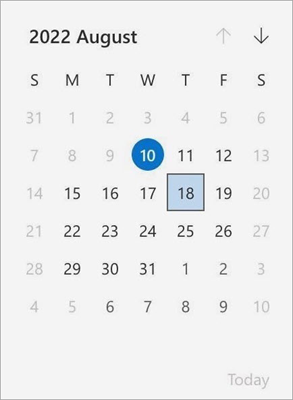This is a cropped screenshot of a calendar page for the month of August 2022. The calendar has a grey background with "2022 August" displayed at the top left corner. Directly below this header, the days of the week are abbreviated and listed horizontally from left to right. The dates of the month are arranged in a standard grid format beneath the days of the week.

Noteworthy elements include:
- The 10th of August, which is highlighted with a blue circle, indicating the current date.
- The 18th of August, which is surrounded by a black box with a light blue fill inside, perhaps marking an important event or deadline.
- The dates from the 10th to the 18th, except for the 13th, are presented in bold black text, suggesting significance or upcoming events.
- Weekend days and past dates are displayed in light grey font, distinguishing them from future weekdays and emphasizing the current date and important future dates.

Overall, this calendar provides a clear and organized view of the month with specific highlighting for current and important dates.